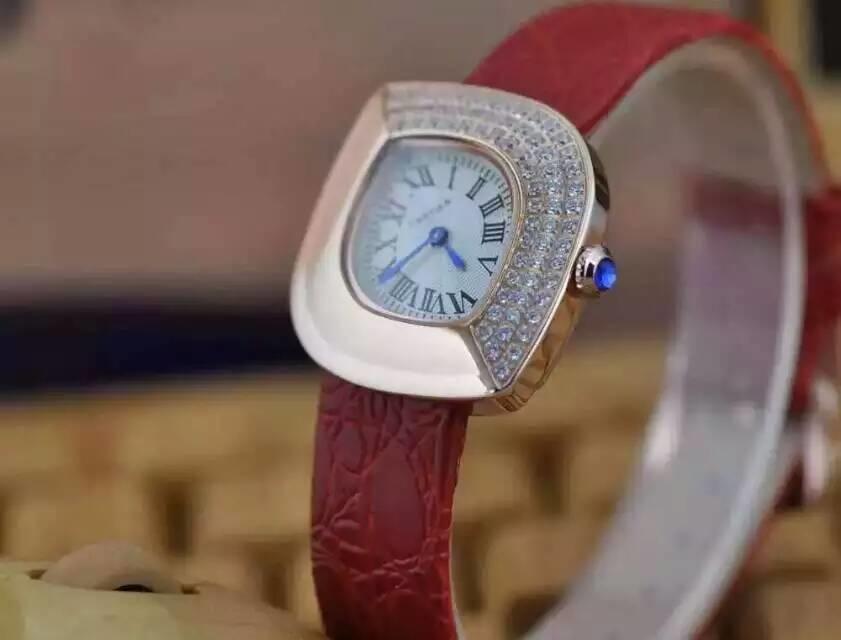This is an indoor, daytime close-up photograph of a wristwatch, showcasing intricate details. The watch features a maroon leather band, adorned with etched designs. The square watch face has a white background with black Roman numerals and blue hands. The perimeter of the watch face is divided into two parts: a silvery section and a gold section, with several white gemstones resembling diamonds set on the gold portion. A silver knob on the right side of the watch is accented with a blue stone in the middle. The left side of the watch is taped with scotch tape. The image has a blurred background with white at the top, transitioning to hints of blue and light brown.